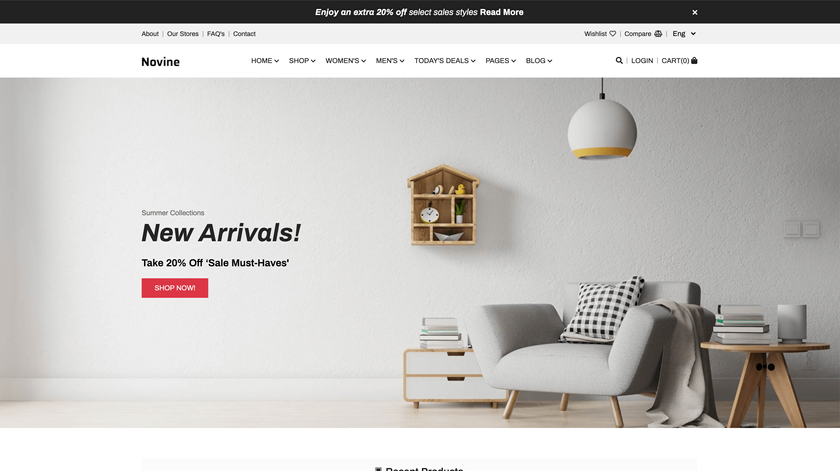The webpage's front page features a sleek, black top border with a promotional banner stating, "Enjoy an extra 20% off select sale styles," accompanied by a "Read More" link. Below this banner, there are navigation links: "About Our Stores," "Frequently Asked Questions," and "Contact."

To the right, there is an options panel including "Wish List" and "Compare," as well as a language selection menu currently set to English. The primary navigation bar includes drop-down menus for "Home," "Shop," "Women's," "Men's," "Tops," "Today's Deals," "Pages," and "Blog." Users can log in via a dedicated button, and the shopping cart icon, currently empty, is also displayed.

The central image showcases a minimalist living room designed predominantly in whites and light grays. A stylish coffee table with books on top stands beside a cozy armchair adorned with a pillow and a throw blanket. Adjacent to this setup is another coffee table with drawers. 

Mounted on the wall is an intricate shelving unit resembling a cross-section of a house, featuring five cubby holes filled with various trinkets and a clock. A chic, oval-shaped hanging lamp, white with a yellow border, is positioned above the armchair. 

Promotional text reads, "Summer Collections, New Arrivals! Take 20% Off Sale Must-Haves," followed by a "Shop Now" call-to-action. The room is painted in an off-white to gray palette, with sleek hardwood floors completing the elegant look.